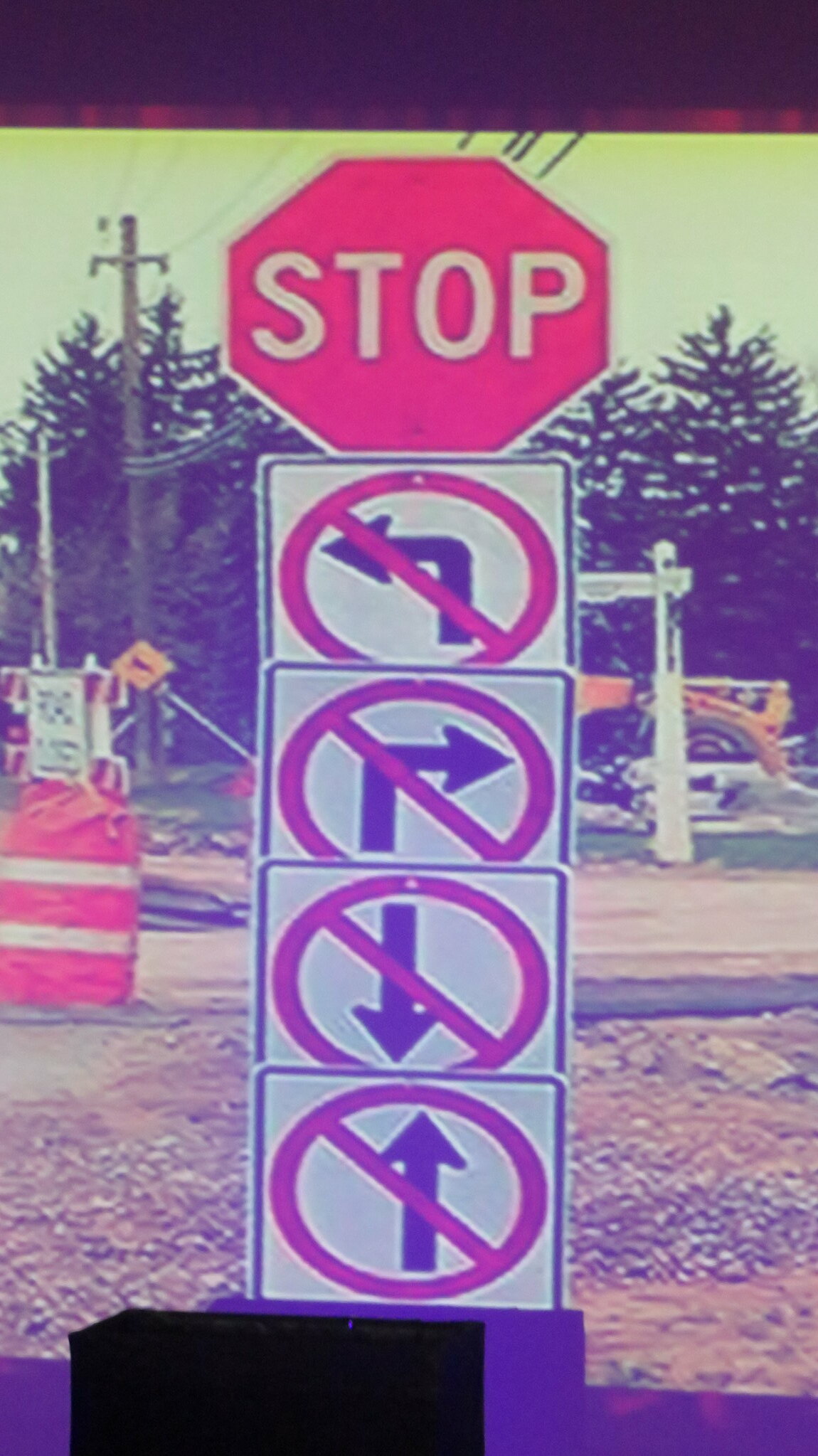In the photograph, a complex construction zone is depicted with multiple cautionary signs affixed below a prominent stop sign. Situated in a sequential manner, the first sign below the stop sign indicates "No Left Turn," followed by a "No Right Turn" sign. Directly beneath these, a third sign showcases a down arrow and an up arrow encircled and crossed out, conveying "No Going and No Coming." In the background, a "Road Closed" sign is visibly placed amidst a terrain littered with gravel and dirt in place of the road. Adding to the scene, an orange construction cone stands near a heavy-duty machine, likely a yellow tractor or grader, indicative of active roadwork.